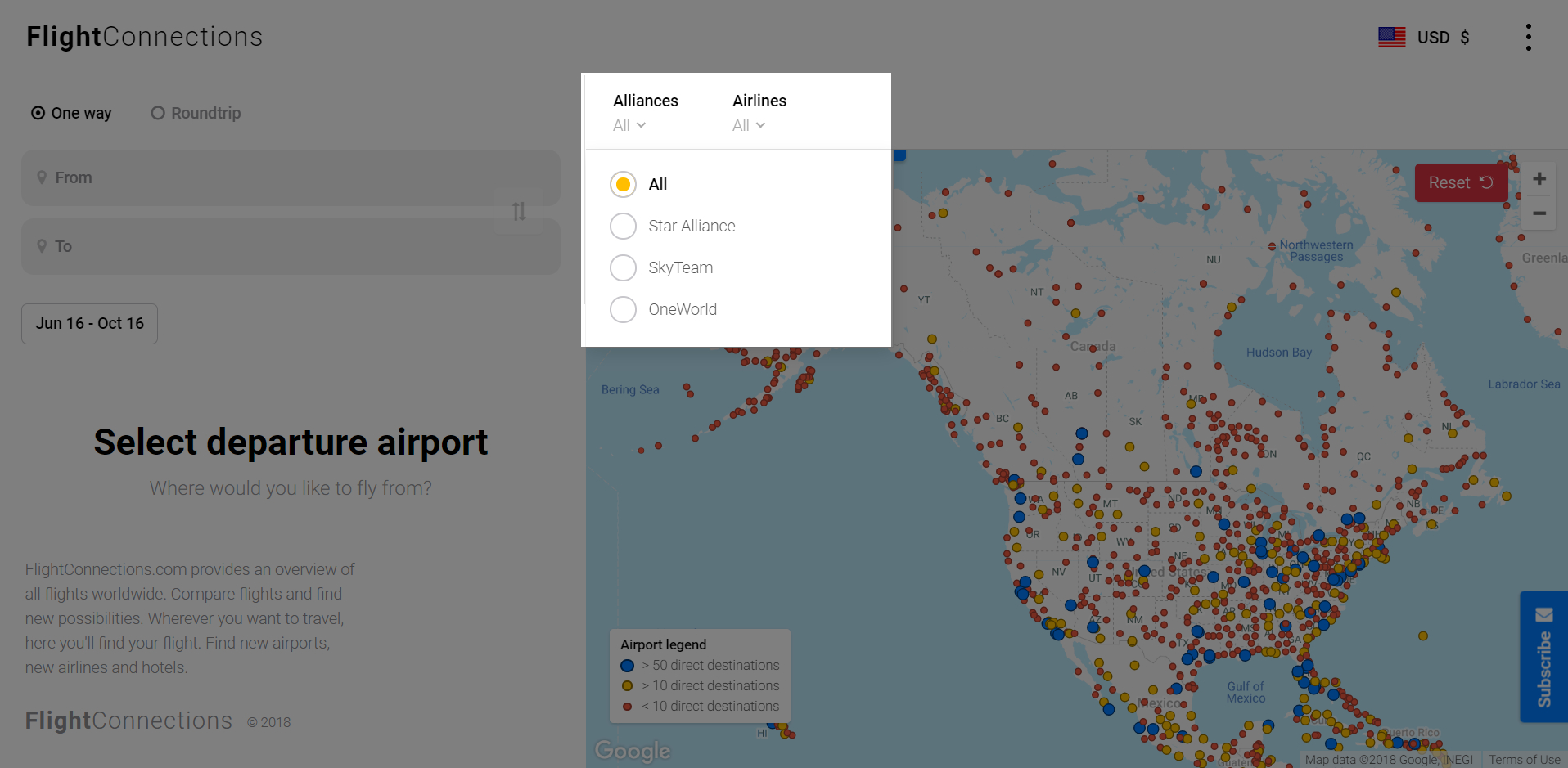This is a cropped screenshot of the Flight Connections webpage. In the top-left corner, the text "Flight Connections" is displayed, with "Flight" in bold typeface and "Connections" in standard font. Below this header, on the left side, there's a panel featuring two horizontal options: "One Way" and "Round Trip," with "One Way" currently selected. Beneath these options are two input boxes labeled "From" and "To," respectively.

Further down on the left panel, there's a small white rectangular box showing the date range "June 16th to October 16th." Below this, centered, is bold black text that reads "Select departure airport." Directly beneath this text, also centered, is a prompt asking, "Where would you like to fly from?"

In the bottom left and right corners, the text explains that Flight Connections provides an overview of all flights worldwide, allows for flight comparisons, and helps users find new travel possibilities, including airports, airlines, and hotels. Additionally, in the bottom left corner, the repeated heading "Flight Connections" appears again.

Towards the center of the page, a small white pop-up box labeled "Alliances" and "Airlines" appears, each with a drop-down menu set to "All." A vertical list of airlines is displayed beneath the pop-up box, with "All" selected.

Dominating the right side of the page is a giant map showcasing hundreds of planes in the air, represented by dots in various colors such as red, yellow, and blue.